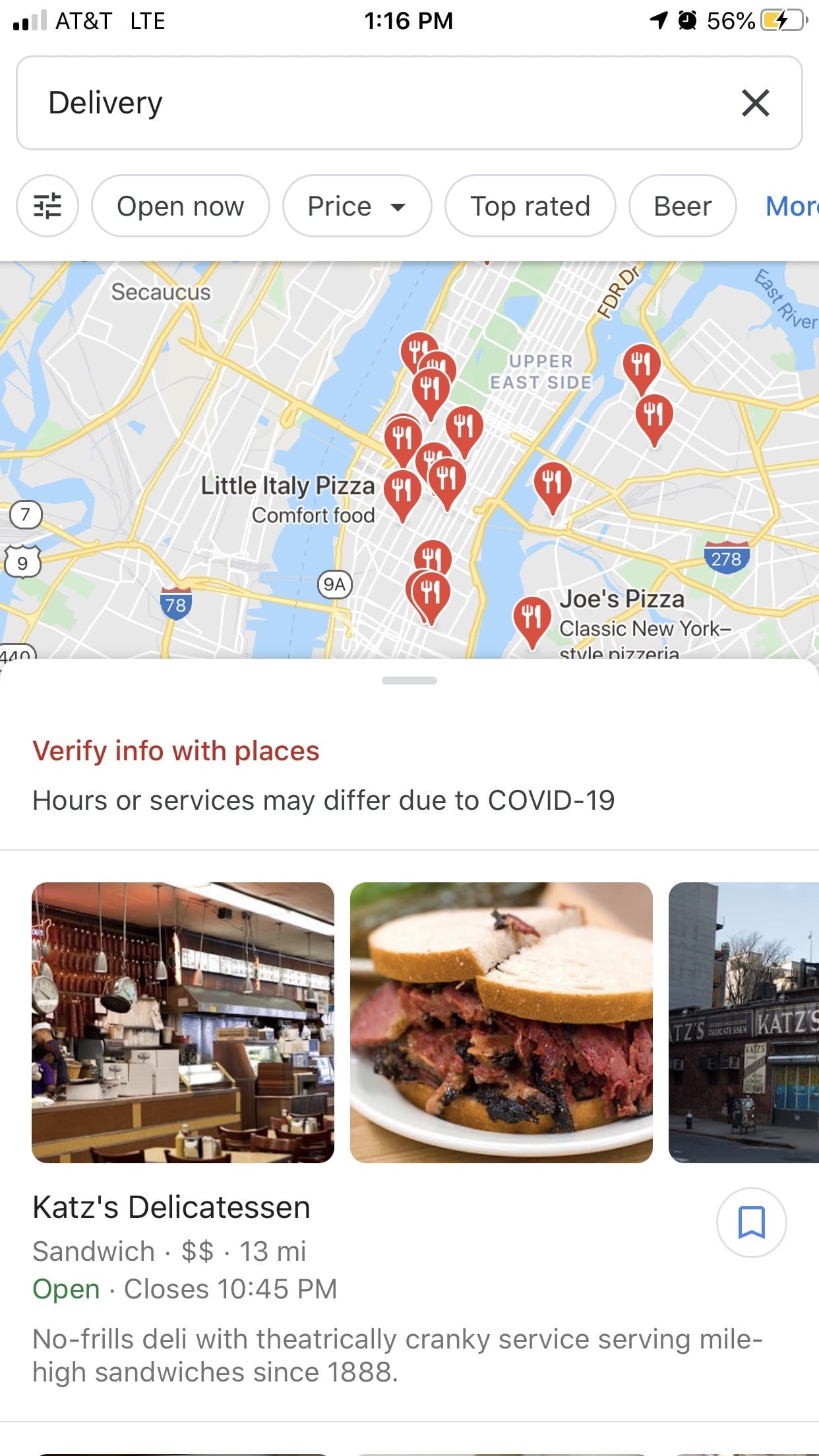The image, captured from an AT&T phone on LTE at 1:16 p.m., prominently displays a partly yellow battery icon with a lightning bolt, indicating the phone is being charged and currently at 56% battery life. The top of the screen shows an alarm clock icon and a delivery notification. The map display includes a heading that recommends popular food destinations such as "Little Italy Pizza" for comfort food, "Joe's Pizza" known for classic New York-style pizza, and "Katz's Delicatessen," famous for its extensive sandwich offerings since 1888.

Displayed on the map are various neighborhoods like Secaucus and the Upper East Side in New York City. Waterways are highlighted in blue, roadways in white, and interstates in yellow. Red pins with fork and knife icons mark restaurant locations across the map. A notification in red advises users to "verify info with places" as "hours or services may differ due to COVID-19."